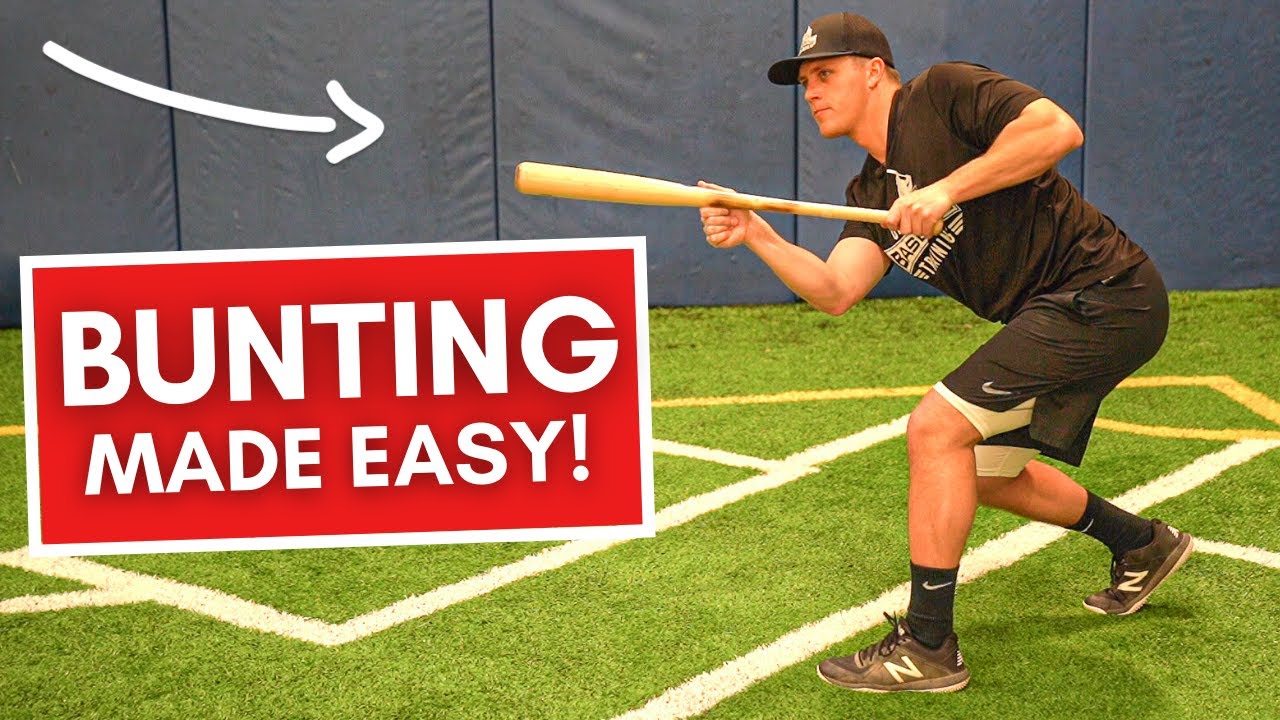The image depicts a YouTube video thumbnail highlighting a bunting demonstration. In the scene, a man dressed in Nike attire, including black shorts, black socks, shoes, and a black hat, is in the act of showing a bunting technique. He is positioned on artificial grass in what seems to be an indoor stadium, adjacent to the protected area next to the stands. The man is bent over, holding a wooden baseball bat with one hand at the bottom and the other near the middle, extending it straight out in front of him. Notably, there are two white lines nearby, potentially marking the pitcher's area. An eye-catching red sign on the left side of the frame reads "Bunting Made Easy" in large, white text, with an arrow pointing to the man's grip on the bat. The overall composition and design elements, such as the text size and colors, suggest that this image is crafted to be a clear and effective thumbnail for YouTube.